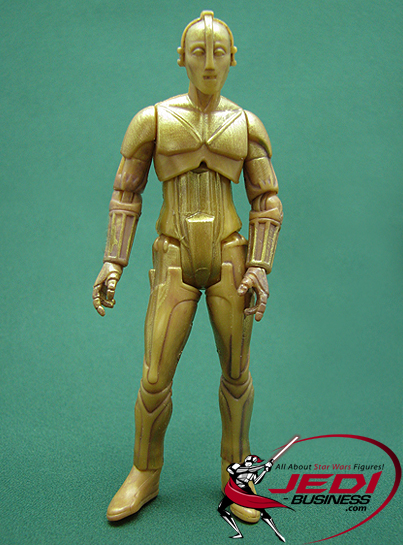The image is an amateurish product photo of a C-3PO action figure. The gold-colored, humanoid robotic figurine, likely made of plastic, has articulable joints for its arms and legs, and stands upright against a green background. Its design, featuring a rectangular mouth, eyelids, and bands crossing over the bald head, does not perfectly mimic the movie character, giving it a somewhat less realistic, more man-like appearance. Below the figure, there's a watermark for JediBusiness.com, with red and black text proclaiming "All about Star Wars figures." In the bottom right corner, there's an additional image of a black-and-white figure with a red cloak and a lightsaber.